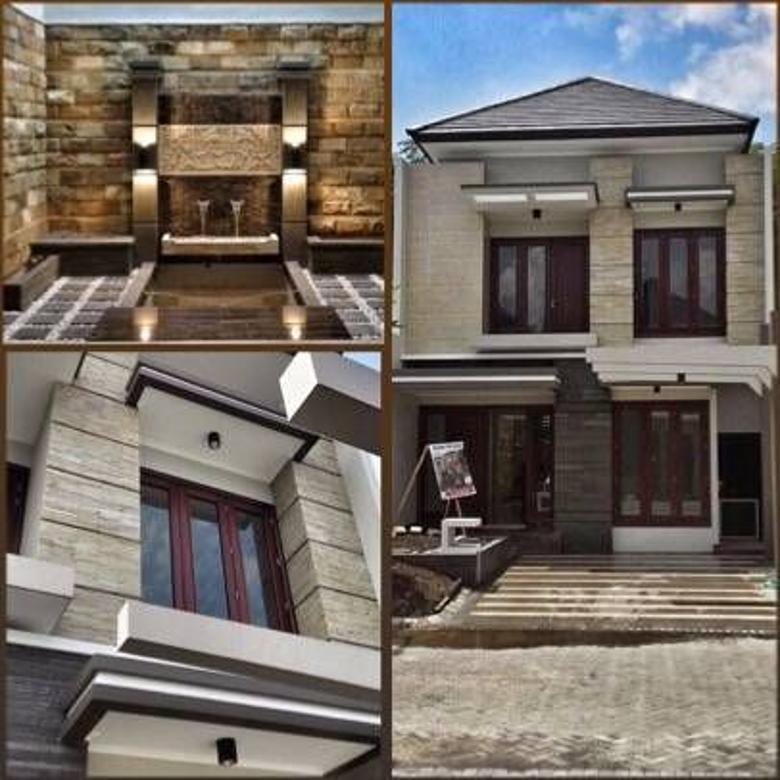This image is a detailed real estate listing featuring a modern, multi-level brick house with a unique and striking architectural style. On the right half of the image, the front facade of the house is displayed, showing a blend of light and dark-colored stone with sections of white-painted areas. The house features narrow sets of windows framed by dark wood, and each window has dedicated outside lighting for nighttime safety and privacy. A visible easel with a poster—likely depicting the realtor—is positioned prominently, hinting at an open house or a property viewing event.

The left upper corner highlights an interior feature: a room with tan brick walls, metallic columns flanking a fireplace mantelpiece, and a uniquely patterned tile floor, suggesting this space is one of the home's standout features. The lower left corner offers a close-up of the narrow, wood-framed windows, showcasing their architectural details, including visible hinges and exterior lights. Overall, the images collectively portray a sophisticated, well-appointed home designed for modern living, blended with artistic architectural elements, suitable for promotional materials on a realty website or brochure.